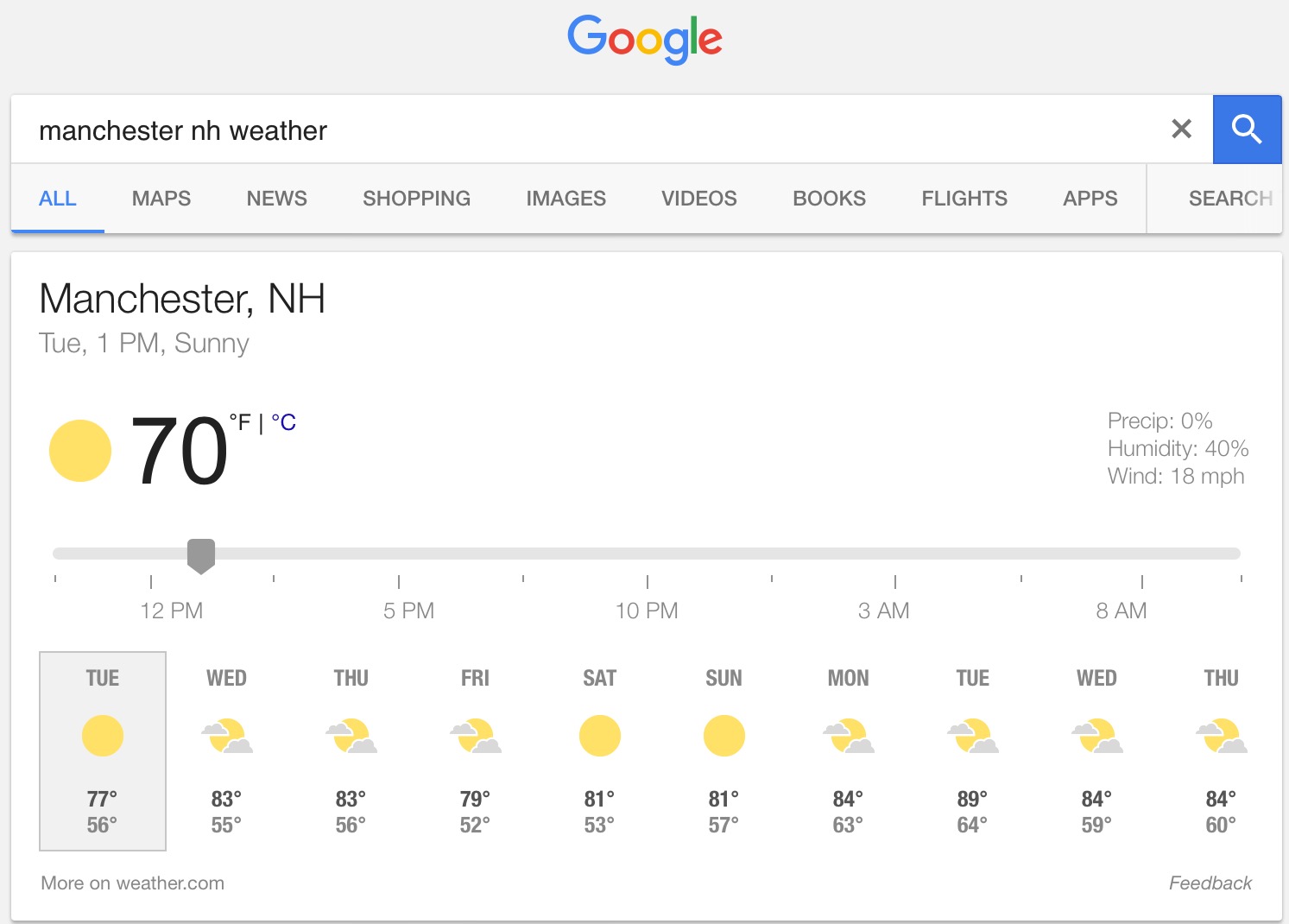The screenshot captures a Google weather forecast result for Manchester, NH. Dominating the top portion of the page is the search bar, which reads "manchester nh weather" in lowercase letters, underneath the centered Google logo. The content area features a prominent white box. In the top left corner of this box, "Manchester, NH" is displayed in large black letters, with "Tuesday 1pm Sunny" noted just below in smaller grey letters. A yellow dot representing the sun appears to the left of "70°F," indicating the current temperature.

Below the temperature, a slider bar extends from left to right, marked with vertical dashes at specific intervals. The times labeled on the bar include 12pm, 5pm, 10pm, 3am, and 8am, with additional dashes present between these markers. At the bottom of the box, a horizontal strip shows the daily forecast. The focus is on Tuesday, but the forecast is available from Tuesday through Thursday of the following week.